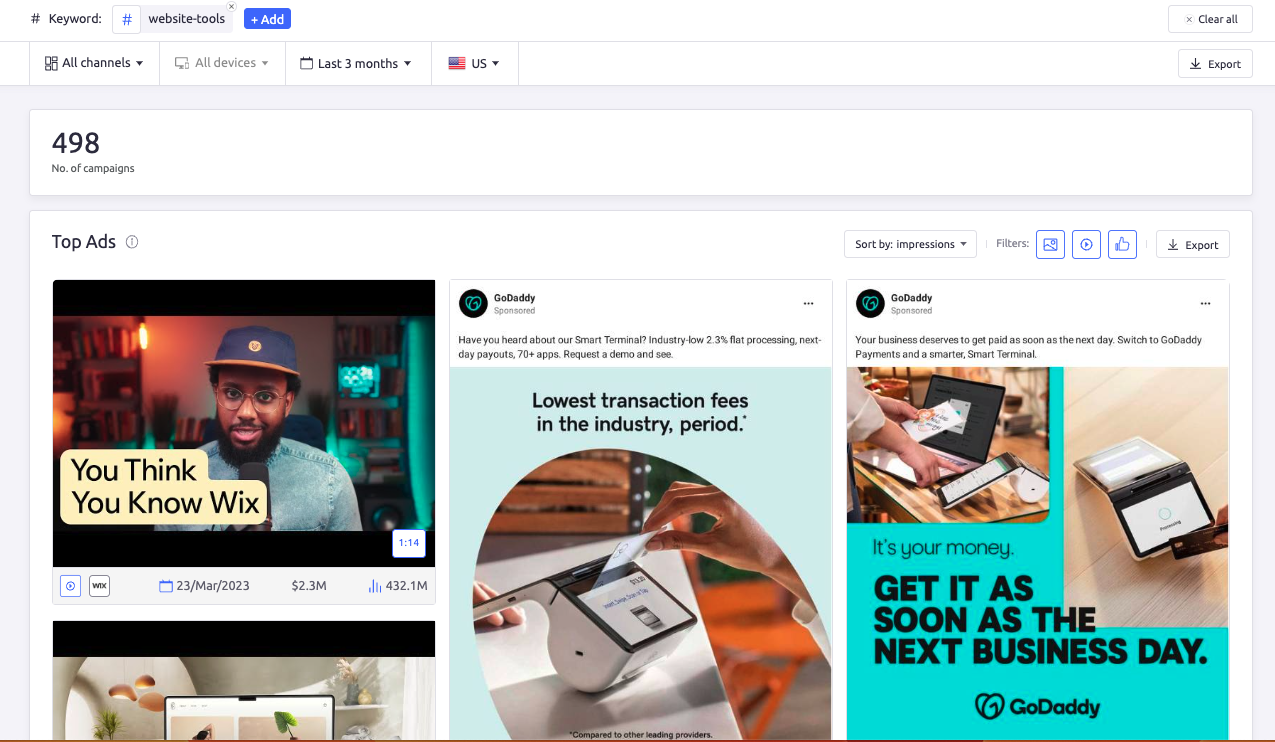The image is a detailed screenshot of a desktop interface, likely related to advertising or marketing analytics tools. At the top left of the interface, there is text that reads "#keyword# website-tools" near a command bar where options to close or add new items are available. The "Add" button is displayed in white text against a medium blue background. On the far right, there is a button labeled "Clear All," marked with an "X."

Below this top section are several dropdown menus labeled "All Channels," displaying various icons, including squares, a smartphone, and a laptop screen. Another dropdown, "All Devices," appears to be grayed out, indicating that it's not currently selectable. The interface also displays segments like "Last 3 months," showing a flag with the text "US."

The next section down reports "498 number of campaigns" and lists numerous ads. Users can sort these by impressions, images, or videos and filter results by the number of likes. There is also an option labeled "Export."

Among the displayed ads, one is for Wix, with the caption "You think you know Wix" accompanied by a 1-minute and 14-second video. The ad is marked from March 23, 2023, and indicates it cost $2.3 million, garnering approximately 432.1 million views.

Another ad, partially cut off, is for GoDaddy, which is identified as sponsored content. The ad reads, "Have you heard about our smart terminal? Industry low 2.3% flat processing fee, next day payout, 70+ apps. Request a demo and see," alongside an image of a device resembling an augmented Apple AirPod with a screen attached. The ad claims "lowest industry fees," with a disclaimer comparing it to other leading providers.

A second sponsored GoDaddy ad states, "Your business deserves to get paid as soon as the next day. Switch to GoDaddy payments and a smarter smart terminal," featuring a man holding a card and a separate image showcasing the terminal with a smartphone and laptop, all promoting the benefits of next-day payouts.

Overall, the screenshot appears to showcase a sophisticated marketing dashboard, offering tools and options to manage advertisements and campaigns.